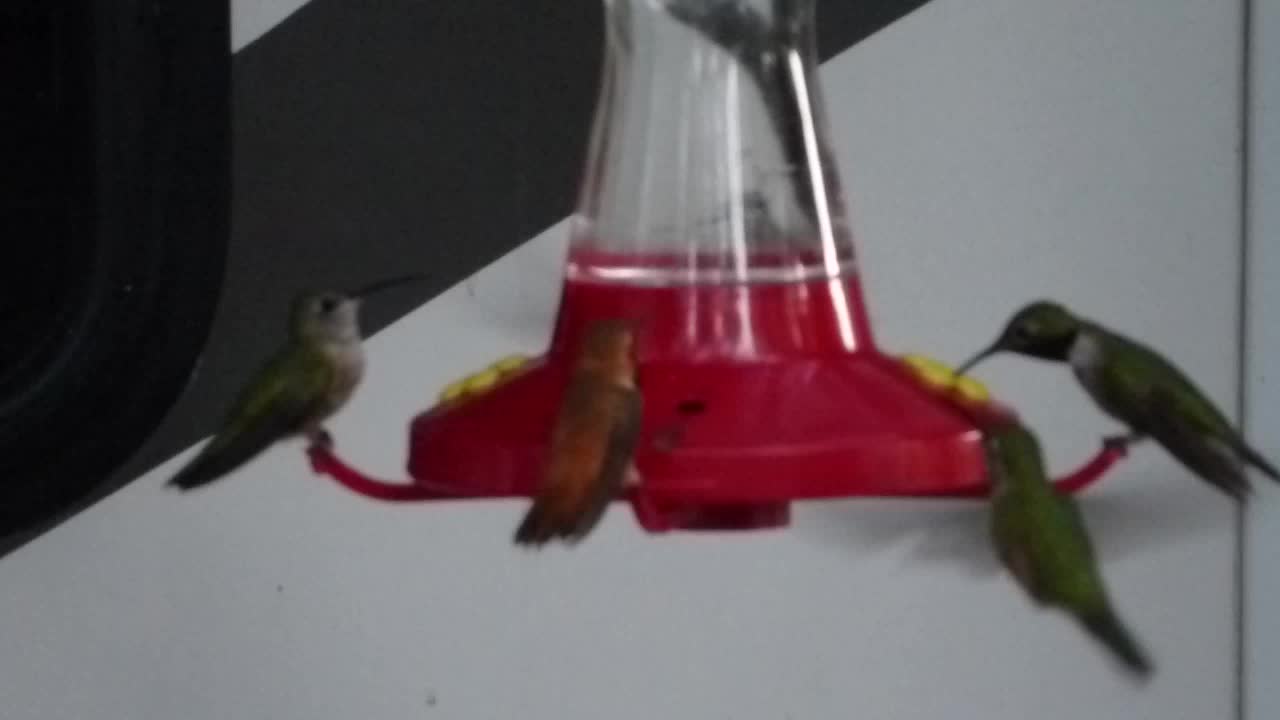The image portrays four small hummingbirds clustered around a hummingbird feeder. The feeder features a bright red base adorned with yellow flower designs, and a clear plastic tube above, likely containing sugar water. The birds themselves display a range of colors: three have green feathers with black tails and beady eyes, while one bird, slightly left of center and still in flight, exhibits a rusty red hue. Due to the limited number of perches on the feeder, the airborne bird appears to be searching for a spot to land. All the birds are poking or attempting to feed at the yellow flowers on the feeder. The image is notably out of focus, suggesting it was taken with a low-quality or old camera, adding to its indistinct nature. The background includes a white wall with a diagonal black stripe, and something black is visible on the left side, making it unclear if the setting is indoors or outdoors.